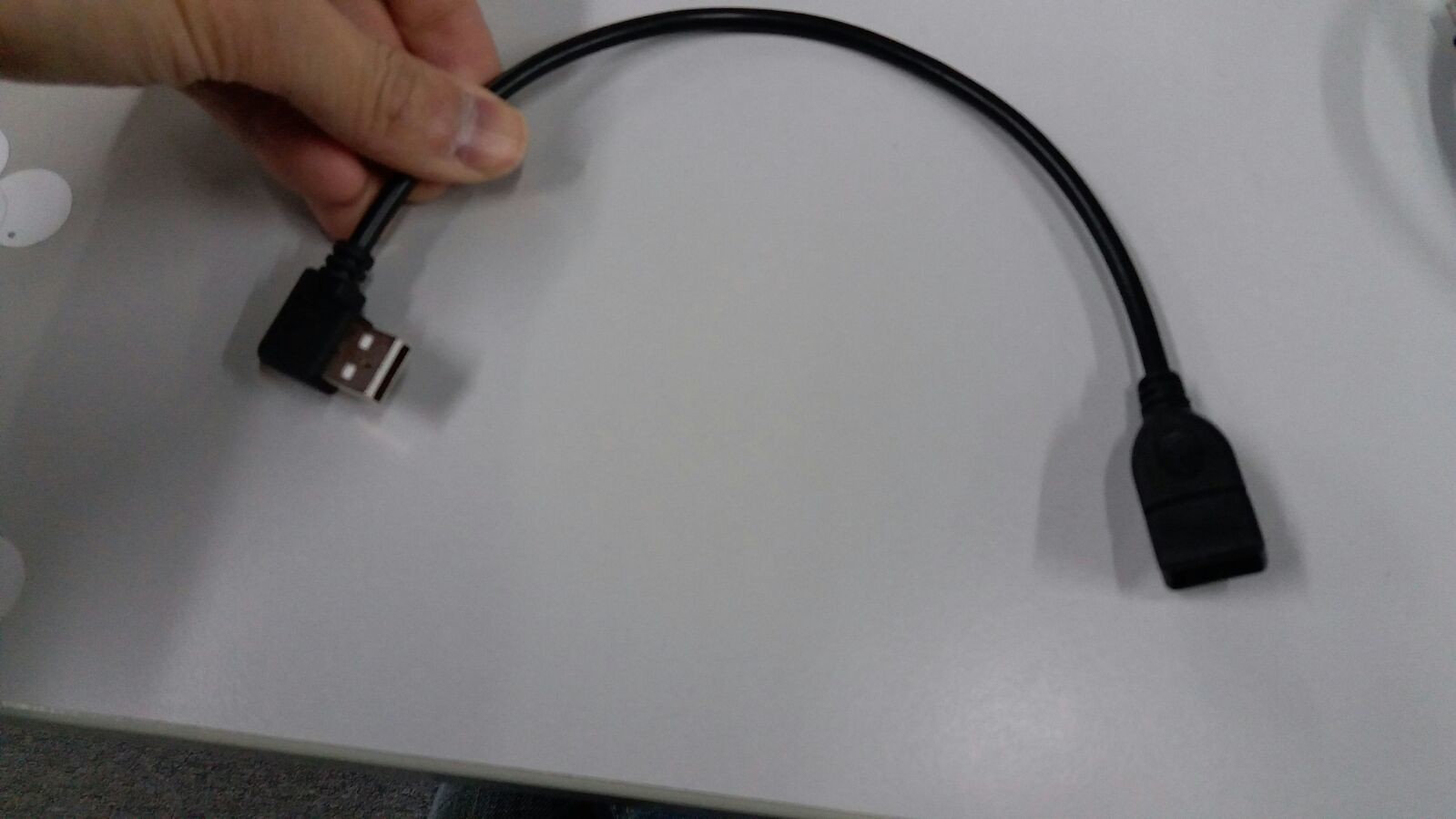The image depicts a close-up of a hand, palm side up, grasping a right-angle USB extension connector. The hand, located in the upper left corner, is holding the black cable between the thumb and four fingers, with part of the wrist visible but partially cut out of the frame. The cable features a male USB plug at a 90-degree angle on one end and extends about six to eight inches to a female USB socket on the other end. The connector appears to be intended for data and video transfer, suggestive of a computer-related work area or classroom setting, characterized by multiple light sources casting varied shadows on a marbly-looking table or light-colored surface dominated by a thick white board-like object.